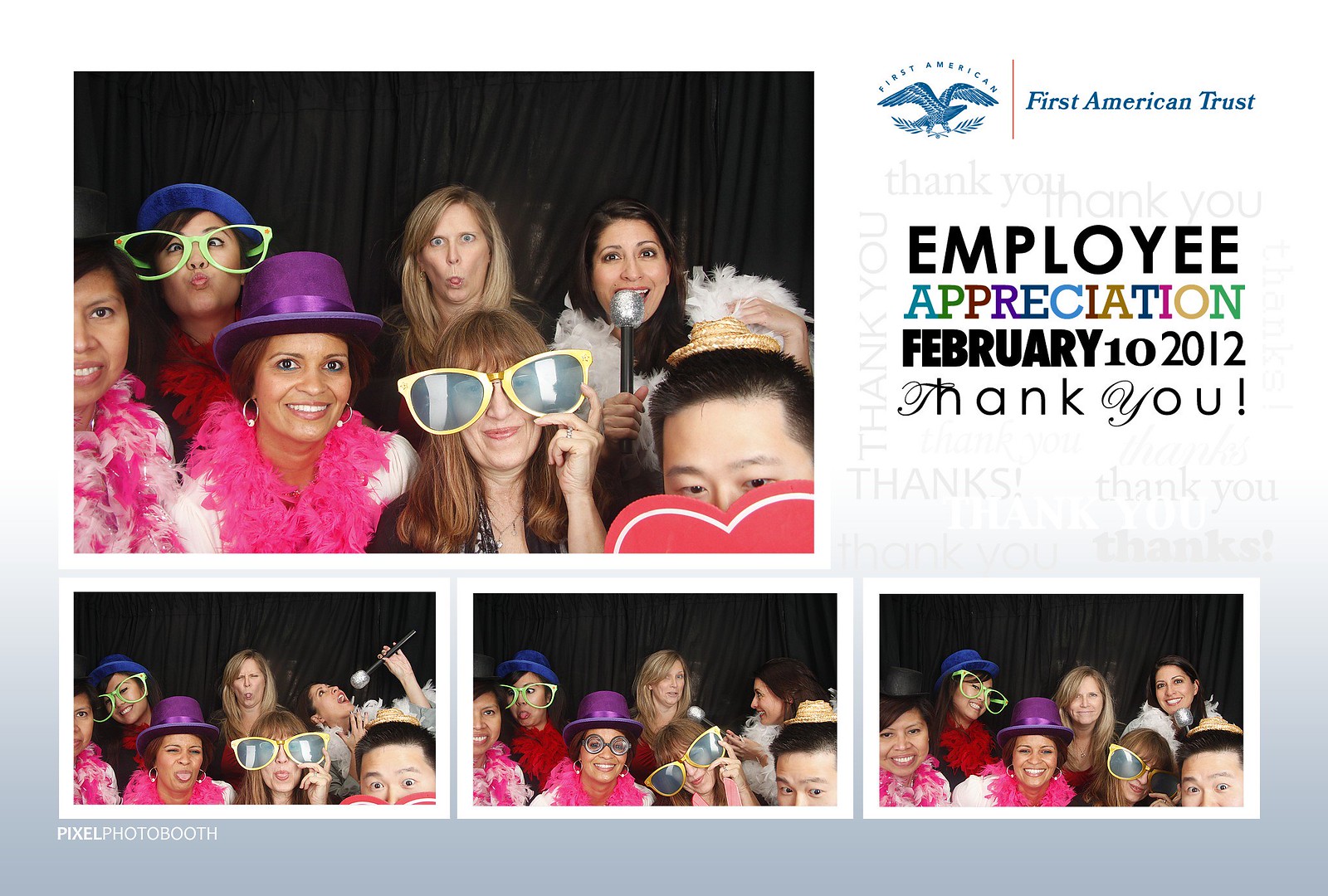This image, styled like a postcard, captures a lively employee appreciation event for First American Trust on February 10, 2012. Positioned in the upper right corner, the text reads "First American Trust" alongside the company logo featuring an eagle, and "Employee Appreciation February 10, 2012" in blue and black text. The word "appreciation" stands out with each letter in a different vibrant color, including shades like blue, green, brown, purple, and more. There are also multiple "Thank You" notes in a light, elegant cursive font. The image itself is a collage featuring four photos: one large at the top left and three smaller ones at the bottom. Each photo shows the same seven employees—six women and one man—wearing wacky props such as green and yellow glasses, blue and purple hats, and other playful items. They're all making fun faces, singing, and dancing, capturing the joyful spirit of the event. The background features a mix of colors like gray, white, pink, and blue, bringing together a vibrant and cheerful scene that emphasizes the camaraderie and fun of the occasion.